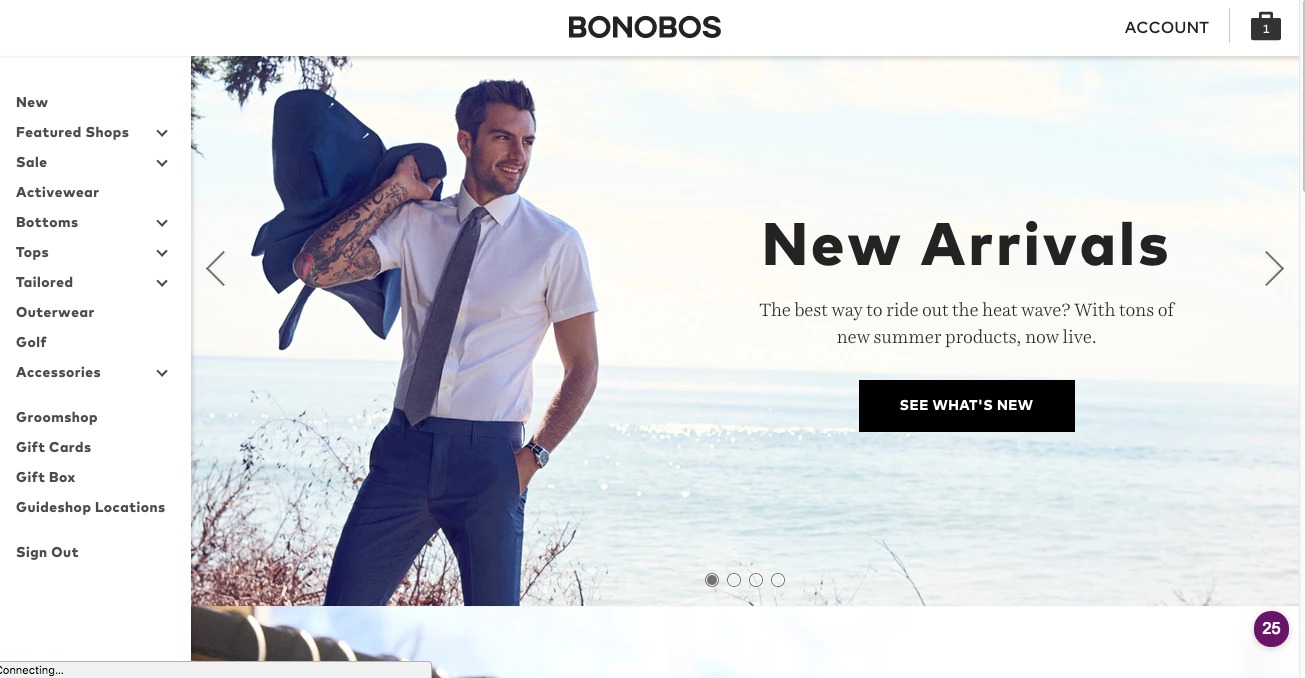The image from the Bonobos website features a stylish man dressed in a white collared shirt paired with a tie, effortlessly tossing a jacket over his shoulder. The backdrop of the image includes a neatly placed "Account" label at the top right corner, alongside an icon of a black shopping bag. Adjacent to the man, a prominent "New Arrivals" sign indicates a fresh collection. Additionally, the caption highlights the phrase, "The best way to ride out the heat wave?" suggesting a seasonal theme. Following this, the text announces the availability of numerous new summer products. A black rectangle with white text at the bottom of the image invites viewers to "See what's new."